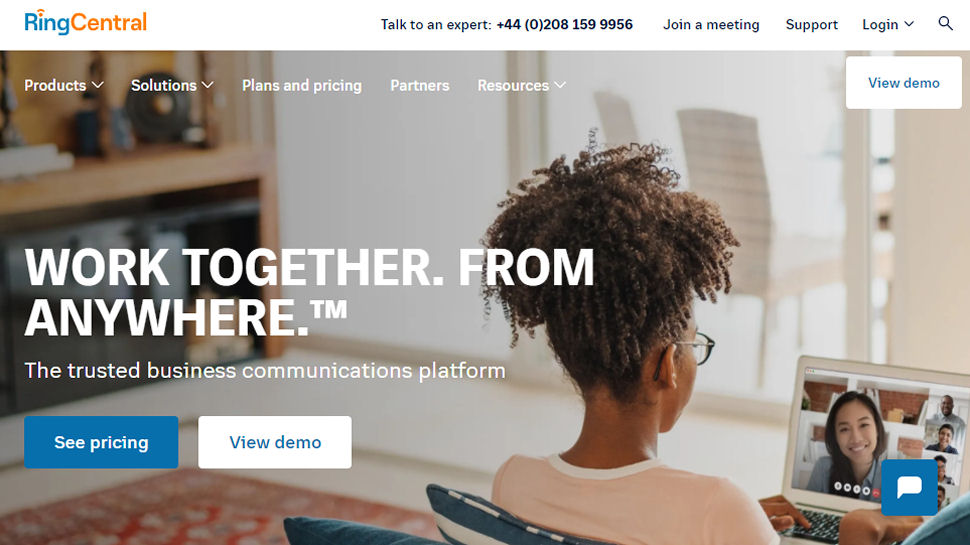In the top left corner of the web page, the logo reads "RingCentral," with "Ring" in bright blue, almost turquoise, and "Central" in orange. The "R" in "Ring" and "C" in "Central" are capitalized, and the dot over the "i" in "Ring" is orange to tie in with "Central." To the right of this logo, there is text in black font that reads, "Talk to an expert:", followed by a phone number. Additional options such as "Join a meeting," "Support," and "Log in" with a down arrow appear, along with a search bar.

In the actual image, which is a horizontal rectangle, slightly to the right of the center, there is a woman viewed from behind. She is seated and wearing a pink shirt. Her glasses are visible as she looks at a laptop. On her laptop screen, a woman is prominently displayed in the main area, while several men appear in a sidebar on the right. The woman is actively typing.

Centered within the image, from the middle of the left edge to slightly past the center, white bold text in all capital letters reads, "WORK TOGETHER. FROM ANYWHERE." Just beneath this text, aligned to the left, are the capital letters "TM." Below that, in sentence case, it states, "The trusted business communications platform."

At the bottom of the image are two buttons. The first button, "See Pricing," is in white font on a blue horizontal rectangular background. The second button, "View Demo," is in blue writing on a white horizontal rectangular background.

Over the woman’s right hand as she types, there is a small blue square with a white speech bubble icon.